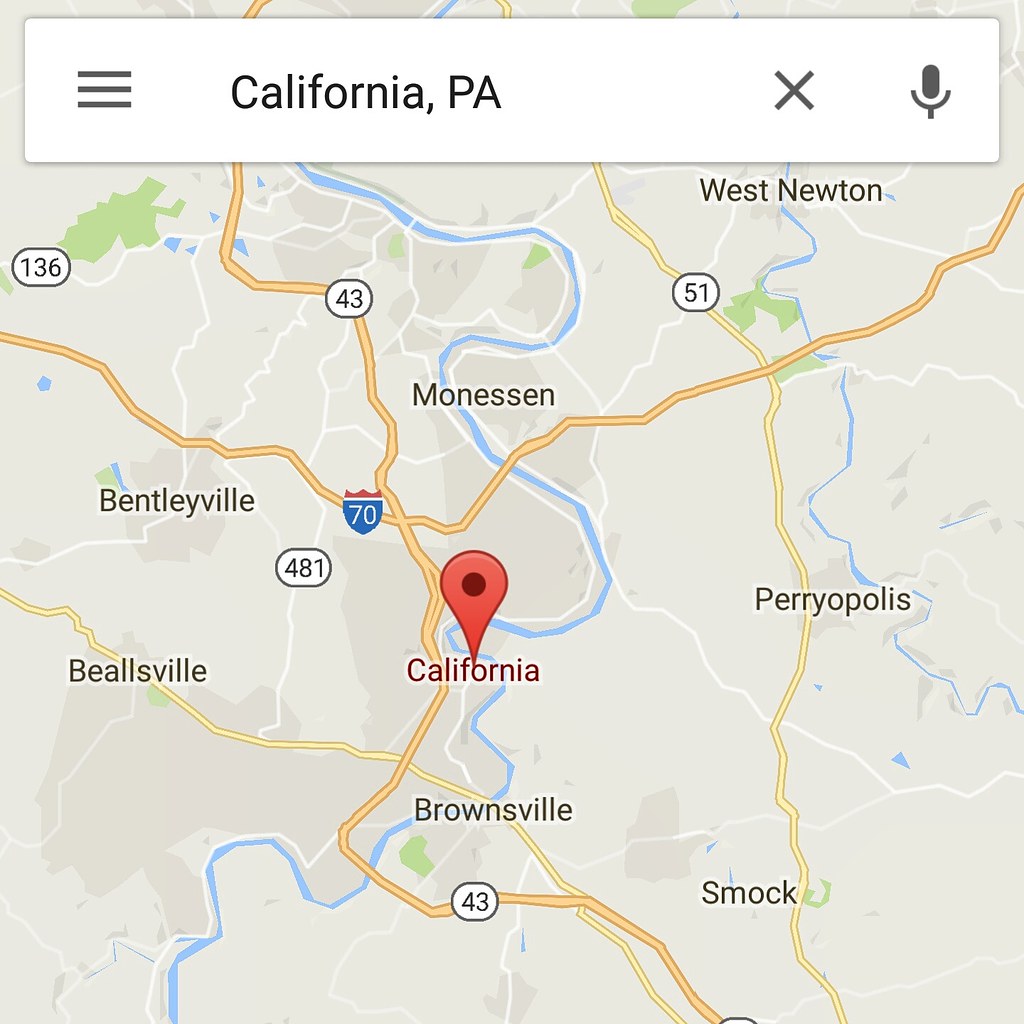The image depicts a digital map, likely sourced from a navigation app such as Google Maps. At the top of the map interface is a white search bar, featuring three horizontal gray lines on the left, a microphone icon on the right, and a gray 'X' positioned adjacent to the microphone. Inside the search bar, in black text, is the location label “California, PA.”

The map itself is predominantly tan with scattered green areas indicating greenery, and blue squiggly lines representing rivers. A red teardrop-shaped marker indicates the specific location of California, PA, with the town name written in burgundy red.

The map also highlights two major routes: Route 43, depicted as a yellow line labeled with the number '43,' and Interstate 70, shown as a yellow line with a blue and red shield icon labeled '70,' situated above Route 43.